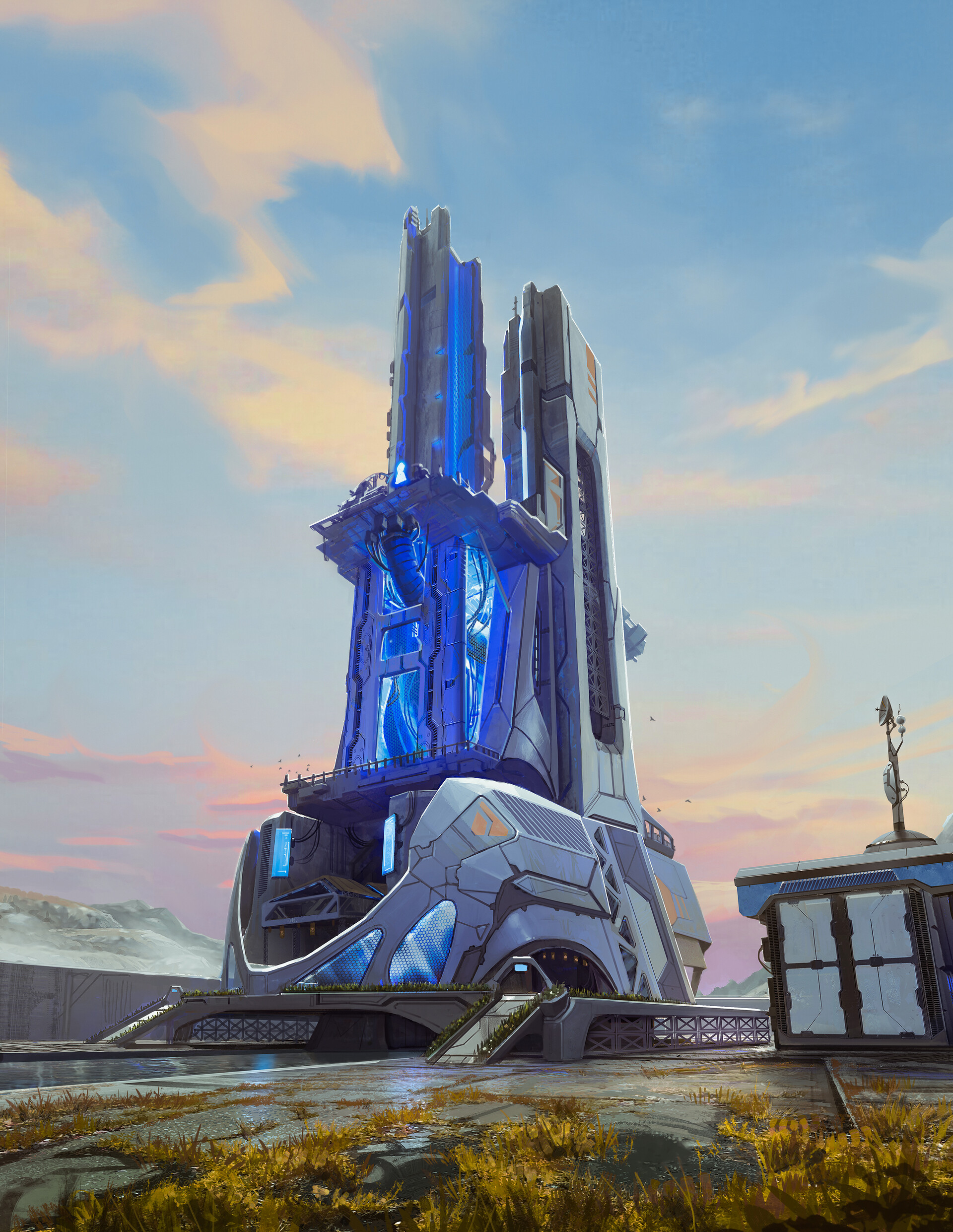This image showcases a futuristic sci-fi power station that resembles a rocket launch pad in an outdoor, modern art setting. The towering structure, which emerges from a concrete pad behind a seawall, is segmented with a jigsaw puzzle-like design and emits blue lights along its metallic columns. The backdrop features a blue sky with minimal clouds and ocean waves crashing against the seawall. At the bottom of the frame, patches of brown grass sprout from cracks in the cemented floor beneath the structure. To the right of this prominent installation, there is a small building adorned with four white squares on its wall and topped with a satellite antenna.